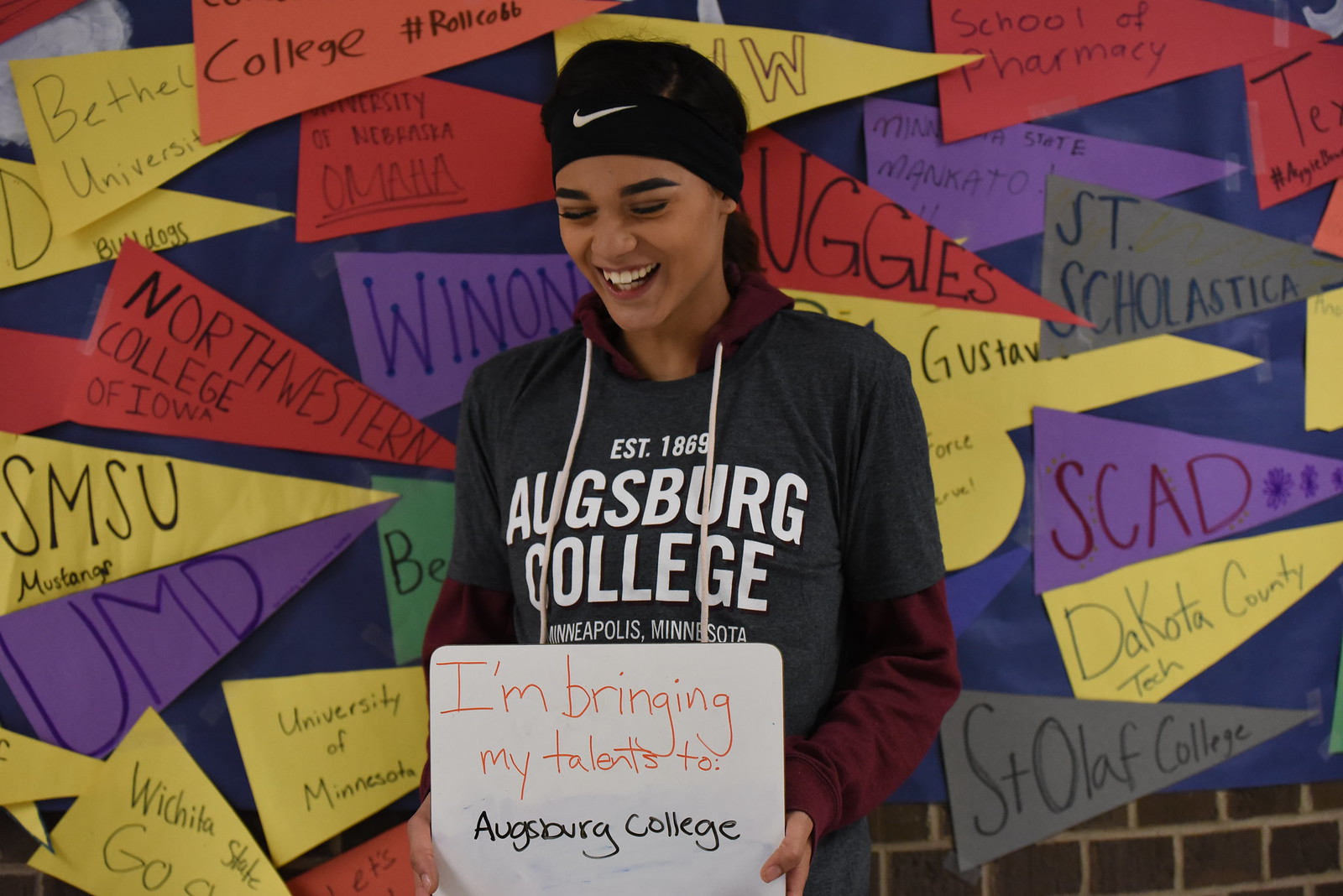The image features a young woman with light caramel-colored skin, dark hair, and a jubilant expression, looking slightly downward with her eyes closed and a wide smile, giving the impression she's laughing. She is wearing a dark Nike headband emblazoned with the iconic white Nike Swoosh. Her outfit includes a greyish t-shirt with white lettering that reads "Augsburg College, Minneapolis, Minnesota," worn over a burgundy hoodie, with the hoodie strings dangling prominently in front. Around her neck hangs a small whiteboard sign with handwritten text in both orange and black lettering, declaring, "I'm bringing my talents to Augsburg College." She stands in front of a brick wall decorated with an array of colorful handmade flags and banners, each representing different colleges with varying colors such as yellow, gray, red, and purple, and featuring names like SMSU, SCAD, and Dakota County. The setting and attire suggest a celebratory moment, possibly related to her athletic commitment to Augsburg College.